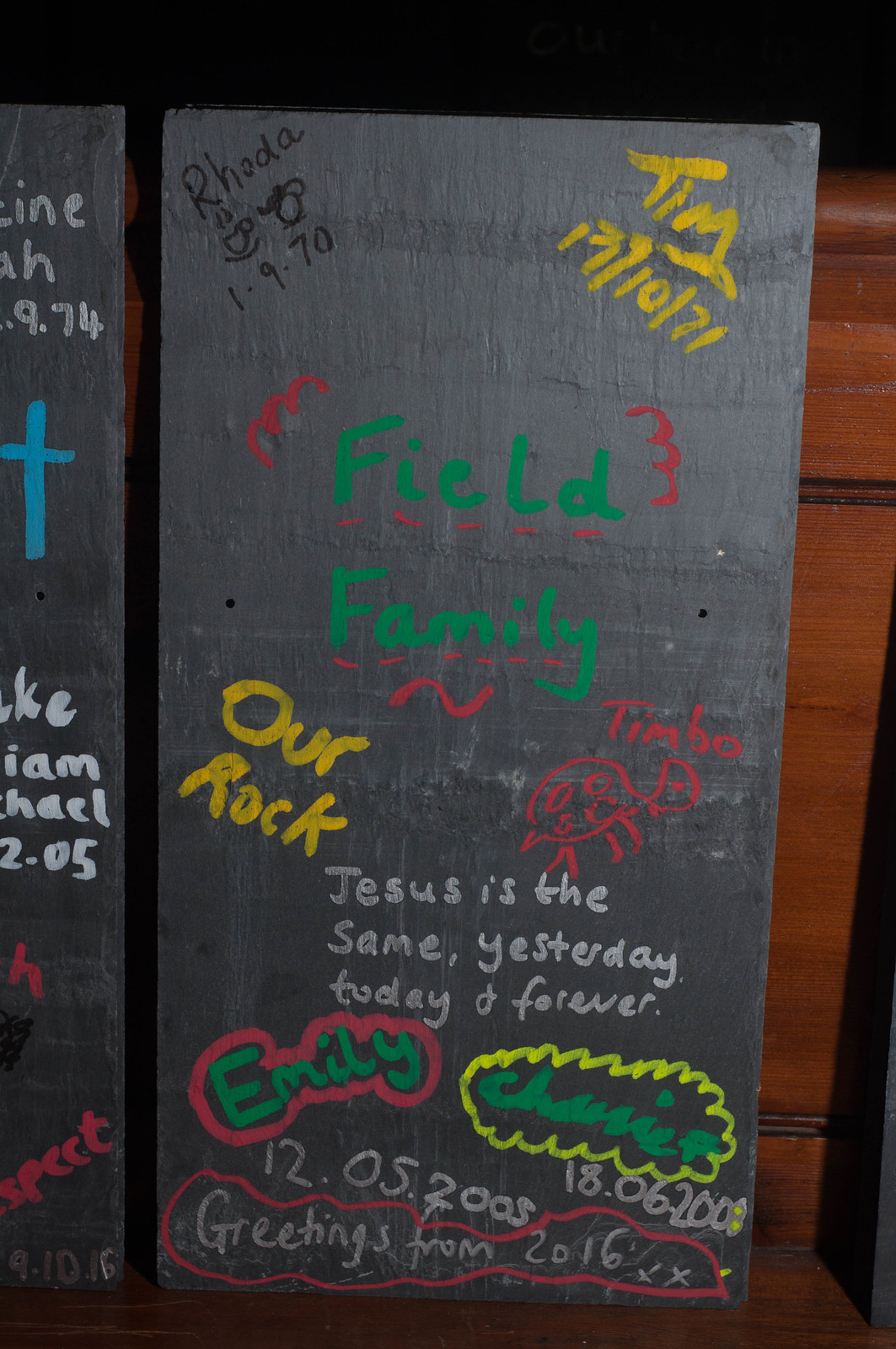The image depicts a series of black, vertical rectangular boards that appear to be slate stone panels or painted boards, resting against a wooden structure, possibly a bench or railing. The primary board in the center features an array of hand-painted text in various colors including green, silver, yellow, and white. The central text reads, "Field Family, Our Rock, Jesus is the same yesterday, today, and forever," with additional names such as Emily and Sherry and the phrase "Greetings from 2016" appearing in different positions. Notable details include "Rota 1970" in the top left corner and "131071" in yellow paint on the top right. The boards are situated in a dimly lit room, with lighting from the right, possibly enhanced by a camera flash captured in the upper right corner of the photograph. The wooden background is visible on the right-hand side and toward the bottom of the image.